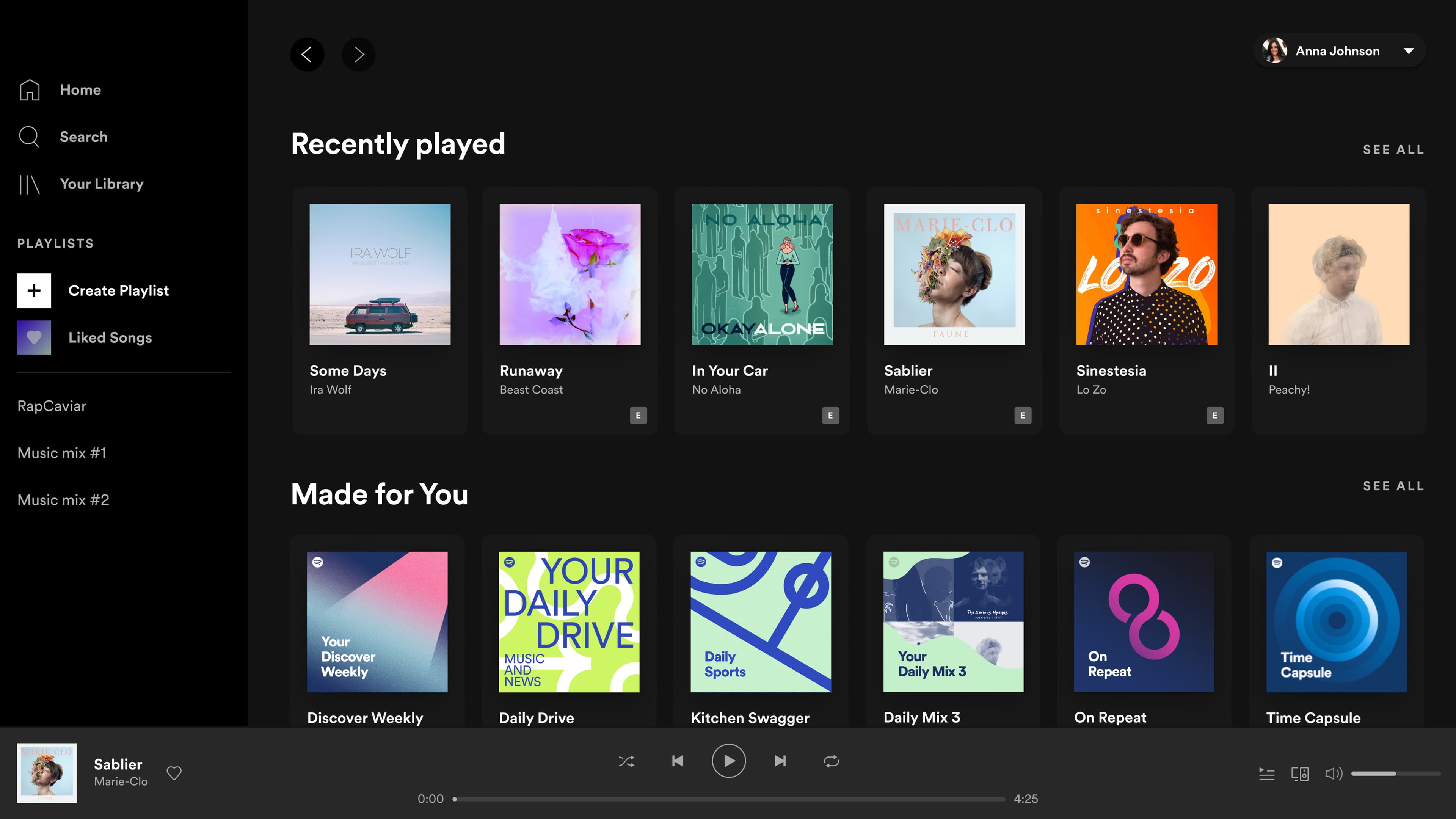A detailed screen capture of a podcast or music app displayed in landscape mode. The user, identified as Anna Johnson, is currently viewing her music account. The left side of the screen features a navigation menu with options including Home, Search, Your Library, Playlists, Create Playlist, Liked Songs, among other unspecified items. At the bottom of the screen, there is a play bar that includes a small icon indicating the currently selected track, along with controls for rewind, fast forward, play, and shuffle functions. The main section of the screen highlights a "Recently Played" area displaying a small album cover and the name of a recently played song. Below that, a "Made for You" section offers personalized recommendations such as "Your Daily Drive" and "Daily Mix," suggesting playlists curated based on the user's listening habits.